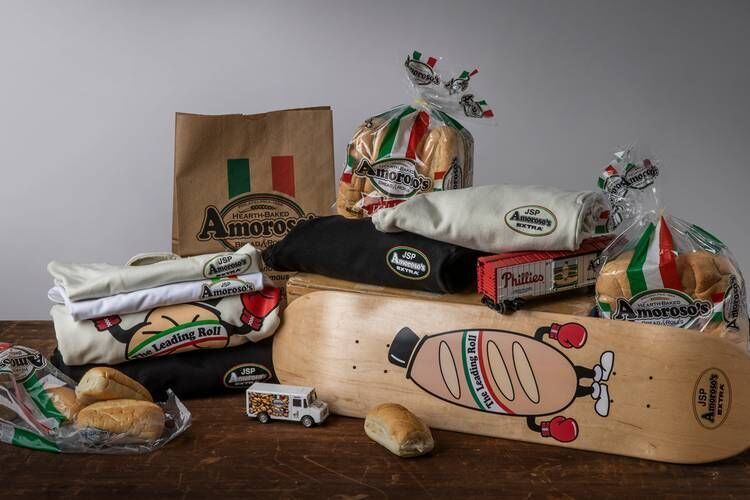The image showcases an advertisement display for Amoroso's bread products arranged on a wooden tabletop against a gray backdrop. Central to the display is a skateboard featuring a cartoon bread roll dressed in a top hat, red boxing gloves, black arms and legs, and white shoes, with "The Leading Role" written across its midsection adorned with red, white, and green bands reminiscent of the Italian flag. Surrounding the skateboard are multiple packages of bread rolls, each marked with the Amoroso’s branding. To the left, a small toy delivery truck and several t-shirts and a tote bag emblazoned with the Amoroso's logo are arranged. A brown paper bag with the same branding is also visible in the background, creating a cohesive promotional setup highlighting the bakery's products and heritage.